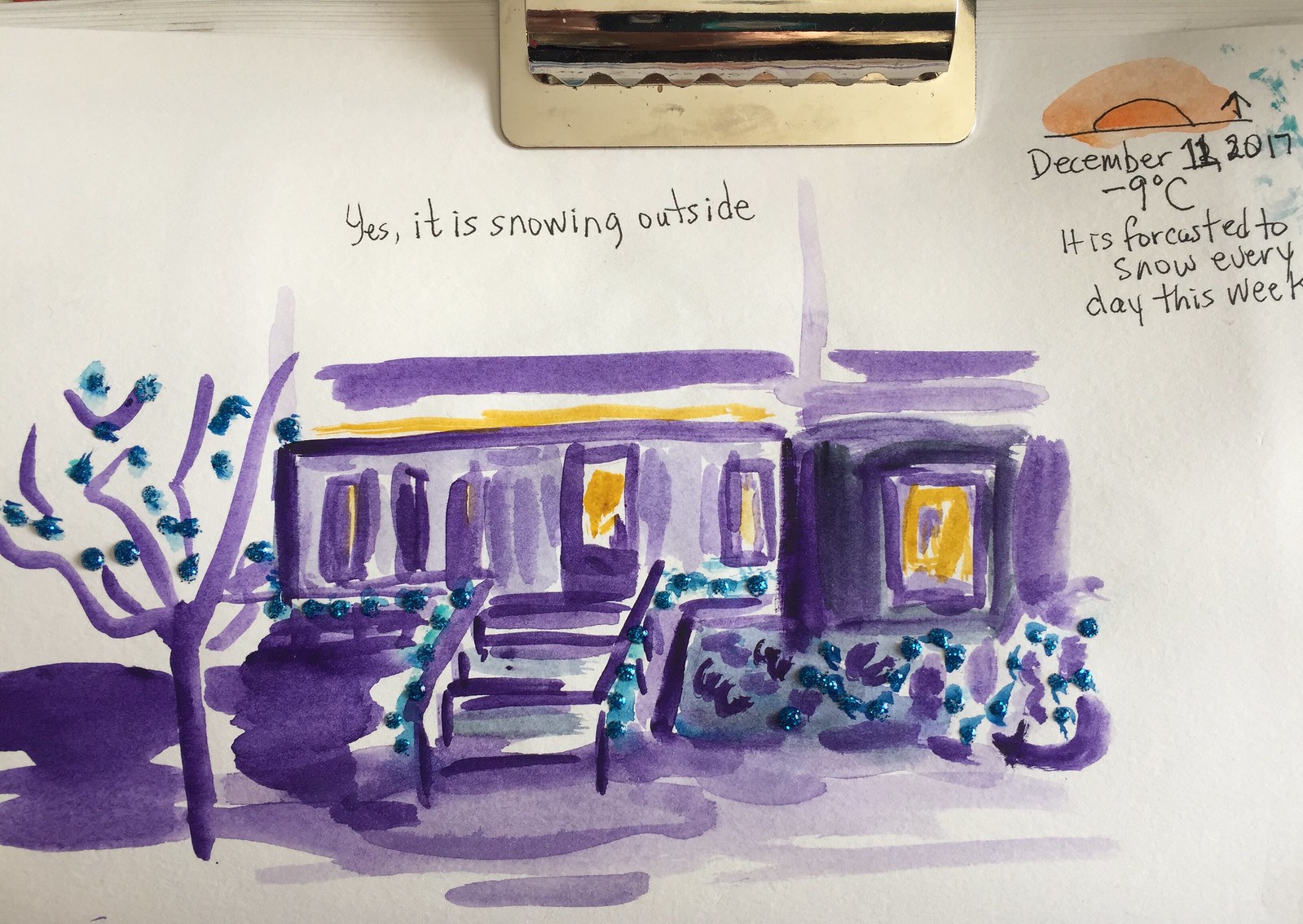This photograph captures a watercolor painting clipped onto a brass clipboard, clearly visible at the top center. Handwritten in ballpoint pen on the white paper, the words "Yes, it is snowing outside" stand prominently. Additionally, in the upper right-hand corner of both the image and the paper, another handwritten note reads: "December 11th, 2017, negative nine degrees Celsius. It is forecasted to snow every day this week." The watercolor painting features a charming depiction of the curb appeal of a house, viewed from the street. The predominant hues in the artwork include purple, blue-green, and yellow, blending harmoniously to create a vibrant scene. Overall, the dominant colors in the entire photograph are white and purple, reflecting the wintry context and the artistic emphasis.